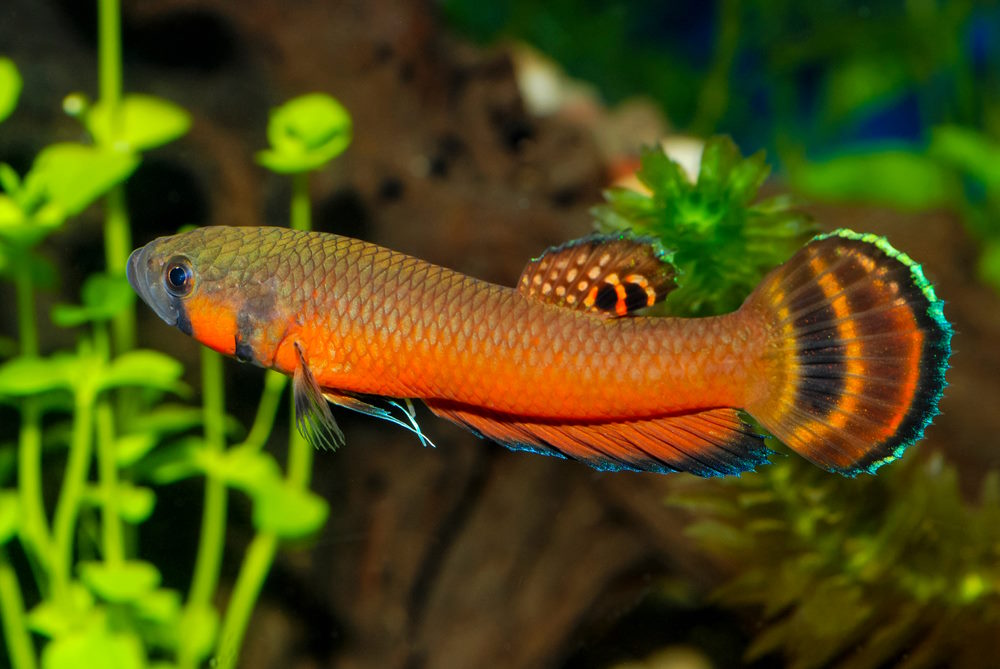This is a close-up photograph of a large, slender fish, strikingly detailed and centered within the frame, seemingly floating against an underwater backdrop of green plant life. The fish's body is primarily a vibrant orange with gold hues on its underside, transitioning to darker, brownish-orange tones along its back. Its mouth area appears grayish, and it has prominent black eyes. The fish's fins and tail are accentuated with intricate patterns and colors—its dorsal fin adorned with speckles of orange and black, and the tips of its fins and tail displaying splashes of blue and hints of neon green. The tail fin features alternating stripes of black, orange, brown, and a touch of iridescent blue-green at the very end. Surrounding the fish are various green plants, some lighter, some darker, with other vague brown elements that blend into the background, which is out of focus. The fish’s scales tessellate in an even diamond pattern running from its head to the tail, adding to its textured appearance. The setting appears to be an aquarium, given the controlled arrangement of plant life and the clear visibility of the fish's intricate details.